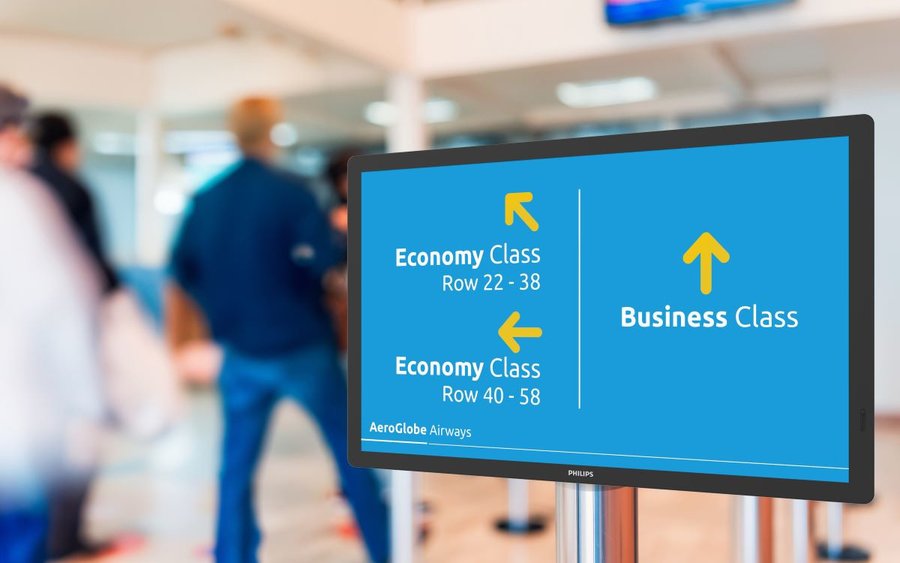This photograph captures a detailed view of a directional sign in what appears to be an airport. The sign is rectangular, light blue with black borders, and mounted on a silver pole. At the bottom of the sign, there is a small Philips logo, hinting that the sign might be a digital display. The sign is divided by a narrow white line. On the left side, two arrows point in different directions for economy class passengers: one arrow points up to the left indicating rows 22-38, and another arrow points directly left indicating rows 40-58. On the right side of the sign, a yellow arrow points straight ahead for business class passengers and another arrow pointing straight ahead indicating AeroGlobe Airways. In the blurred background, a white ceiling and a blue monitor can be seen, along with a line of people likely waiting in line. Among the individuals, one man is wearing a blue shirt and blue pants, while another person behind him is dressed in a white shirt and blue pants, carrying a bag.